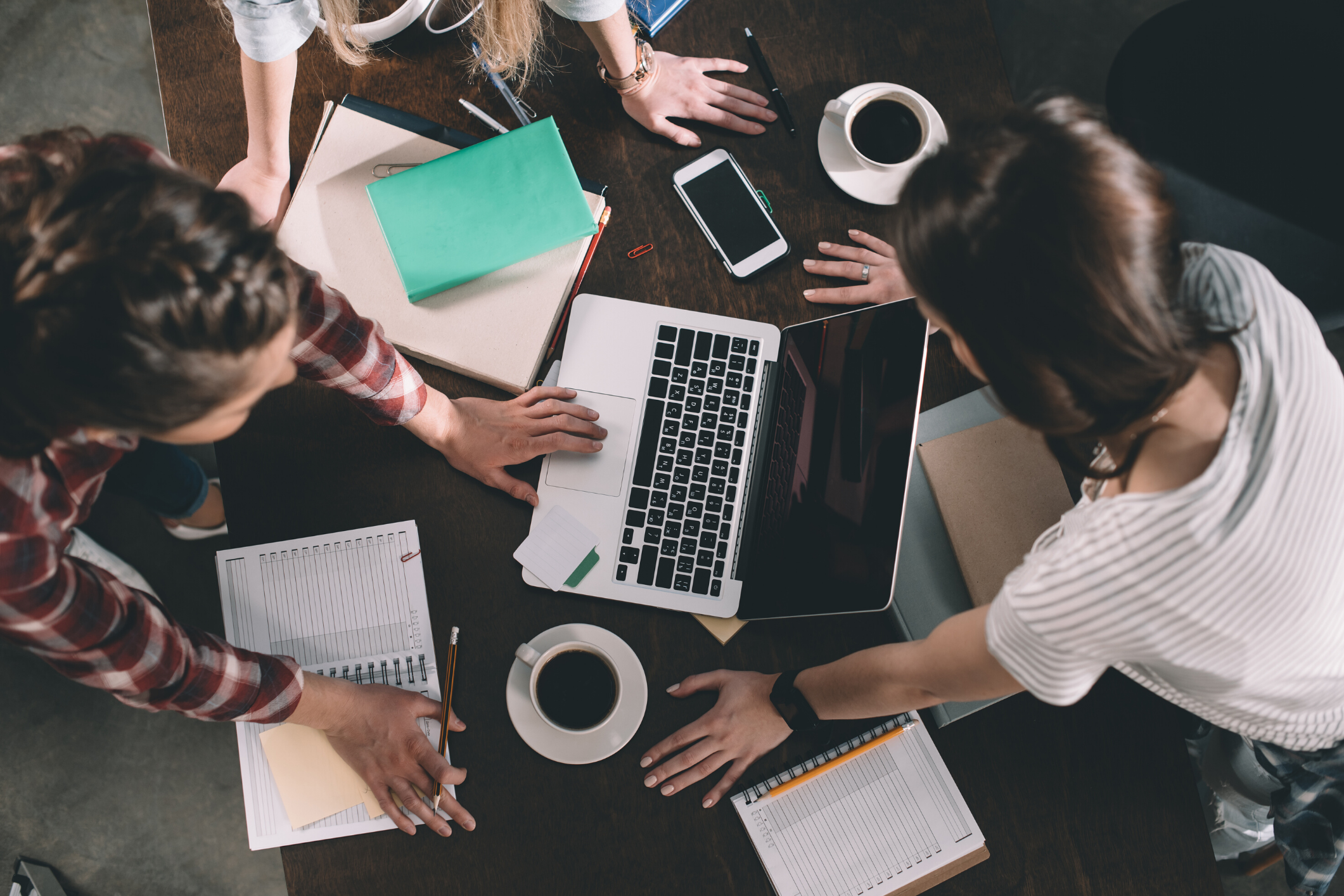This color photograph captures an overhead view of three women leaning over a large, dark brown wooden table, which is scattered with various office supplies. The perspective is like you're standing above them, looking down. Each woman has her hands resting on the table, suggesting they are engaged in a collaborative task.

In the upper left-hand corner, just her hands and long blonde hair are visible, is a woman with a white shirt. In front of her, a tan-covered notebook is topped with a smaller, green-covered notebook. By her left hand, a smartphone with a blank black screen lies next to a white saucer holding a white mug filled with coffee.

Directly in front of the blonde woman and slightly to the right, another woman with short brown hair and a horizontally striped gray and white shirt is visible from the top of her head. Her hands are also on the table, and before her sits a laptop turned towards the blonde woman. This woman appears to be resting her hands on the table.

In the lower right corner of the frame, another woman with dark brown hair is standing. She wears a flannel shirt with dark red, white, and gray stripes, its sleeves pulled up above her wrists. Her hands rest on the table with a pencil in one of them, focusing on the same laptop. Around her lies a variety of notebooks, and near her is another white mug on a white saucer filled with coffee.

This image captures a sense of focused collaboration among the women, likely in their 20s or early 30s, as they work together around the table, surrounded by notebooks, a laptop, and coffee, indicative of a productive office or study session.